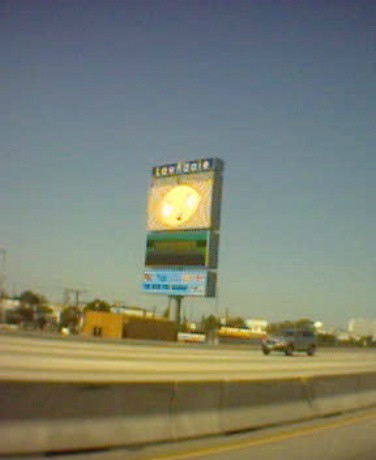A vertical image depicting a somewhat blurry urban scene under a bluish-gray sky with an ombre effect. The sky transitions from a darker blue-gray at the top to a lighter shade towards the horizon. Below, a road is visible with a median dividing traffic directions. Large billboards rise on sturdy posts, though the advertisements are indiscernible due to the image's lack of clarity. A single car can be seen traveling to the left. Power lines stretch across the background, and various buildings are present, adding to the urban landscape. Despite the blur, the overall context of the scene remains identifiable.